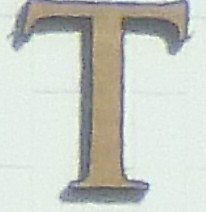The photograph depicts a somewhat blurry, zoomed-in image of a sign from a distance. At the center of the image is a single, capital letter "T" rendered in a standard serif font, possibly reminiscent of Times New Roman. The letter appears to be a 3D object made of material with earthy brownish tones. It casts a slanted shadow to the left, suggesting it is outside and part of a building's facade. The background is a light greenish off-white wall that seems to be constructed from a concrete-like material. The overall setting suggests the letter "T" is part of a storefront sign or similar architectural feature.